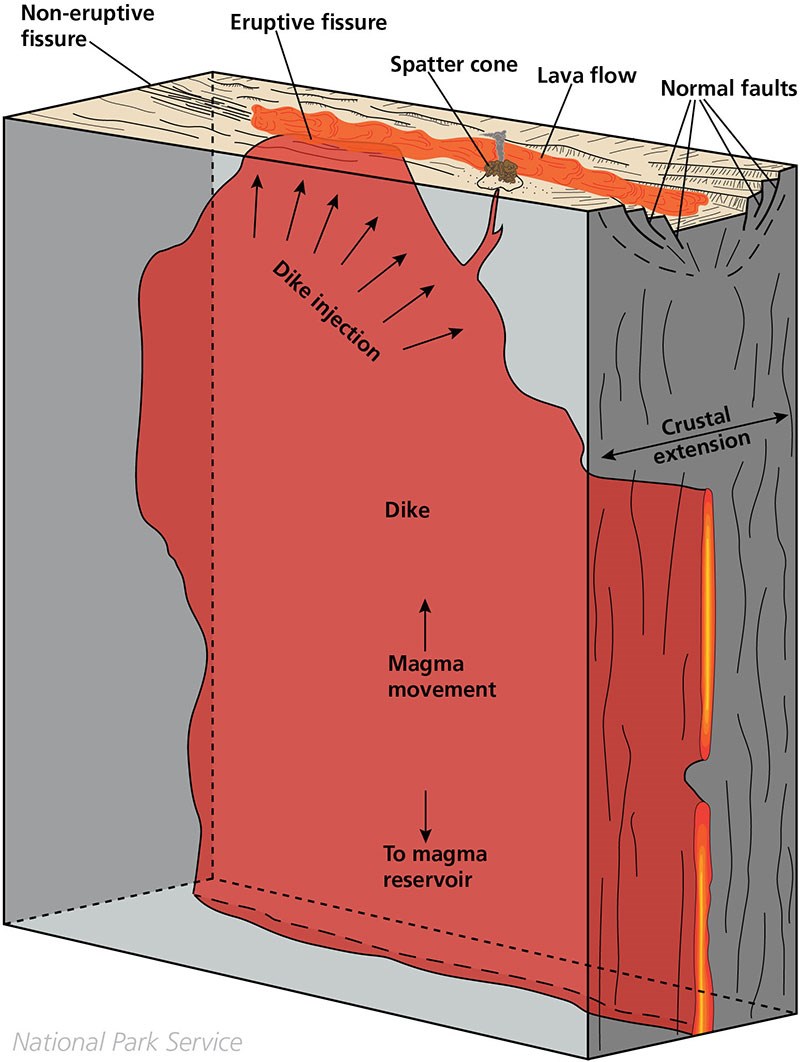The image, provided by the National Park Service, is a detailed diagram depicting the movement of magma beneath the Earth's surface. The diagram shows a cross-sectional view, where the top part represents the earth's surface and the bottom part illustrates various subterranean features. Dominating the lower section is a red-colored area labeled "dike," where multiple arrows indicate "dike injection" directing magma upwards. Further down, arrows point to a "magma reservoir" and highlight "magma movement" towards the surface. 

The top of the diagram illustrates several geological features: "non-eruptive fissures," "eruptive fissures," "spatter cone," "lava flow," and "normal faults." These elements depict different volcanic and tectonic activities. The term "crustal extension" appears beside the diagram, emphasizing the horizontal stretching of the crust. Overall, this comprehensive diagram effectively explains the process by which magma rises from deep within the Earth to the surface, causing various geological formations and activities.